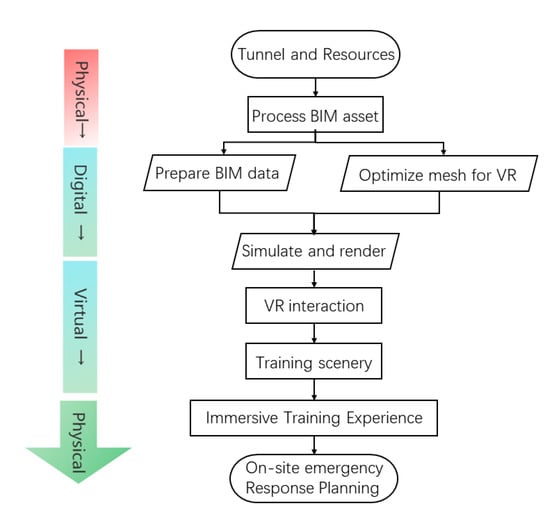The image is a detailed flowchart, potentially from a tech manual, illustrating the transition from physical to digital, virtual, and back to physical. On the far left, a vertical arrow indicates these stages: physical, digital, virtual, and physical. To the right of this arrow, the flowchart begins at the top with "Tunnel and Resources," followed by an arrow pointing down to "Process BIM Asset." This node splits into two branches: the left branch indicates "Prepare BIM Data," while the right indicates "Optimize Mesh for VR." Both branches then converge at a single point labeled "Simulate and Render." From this point, the flow proceeds downward through several stages: "VR Interaction," "Training Scenery," "Immersive Training Experience," and finally "On-Site Emergency Response Planning."